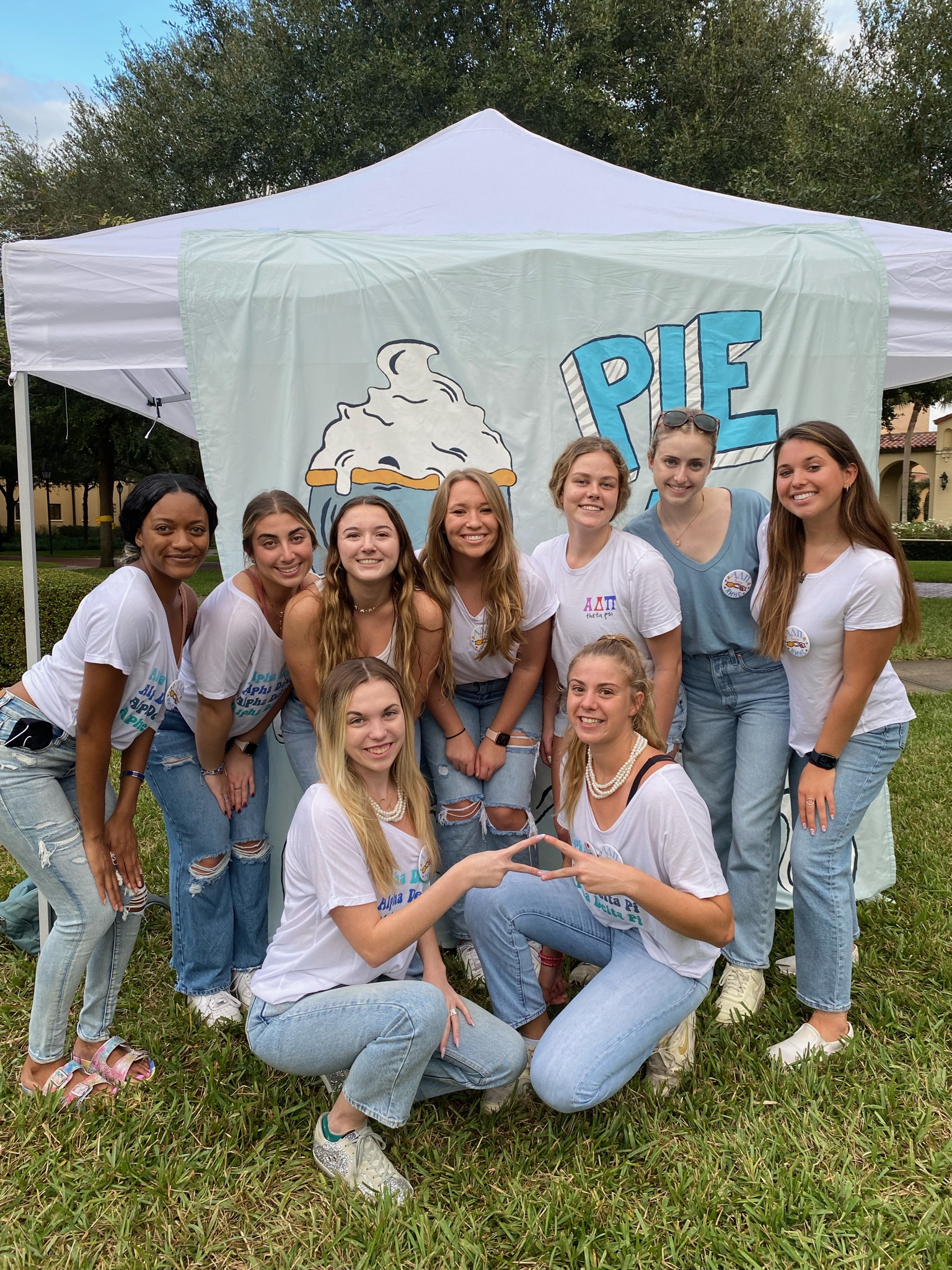The image features a group of nine sorority sisters from Alpha Delta Pi posing for a group photo in a grassy area, likely on a college campus. They are all dressed in casual attire, wearing white t-shirts and various shades of blue jeans, with most of them sporting white shoes. Seven girls stand in the back row while two are crouching in the front, forming a traditional college fraternity hand signal. The diverse group includes a mix of ethnicities, with several brunettes, blondes, and one African American woman. The background showcases a canopy with a banner that prominently displays the word "pie" along with an image of a pie. Beyond the canopy, part of a building and some trees are visible, suggesting an outdoor event, possibly a sorority fundraiser.